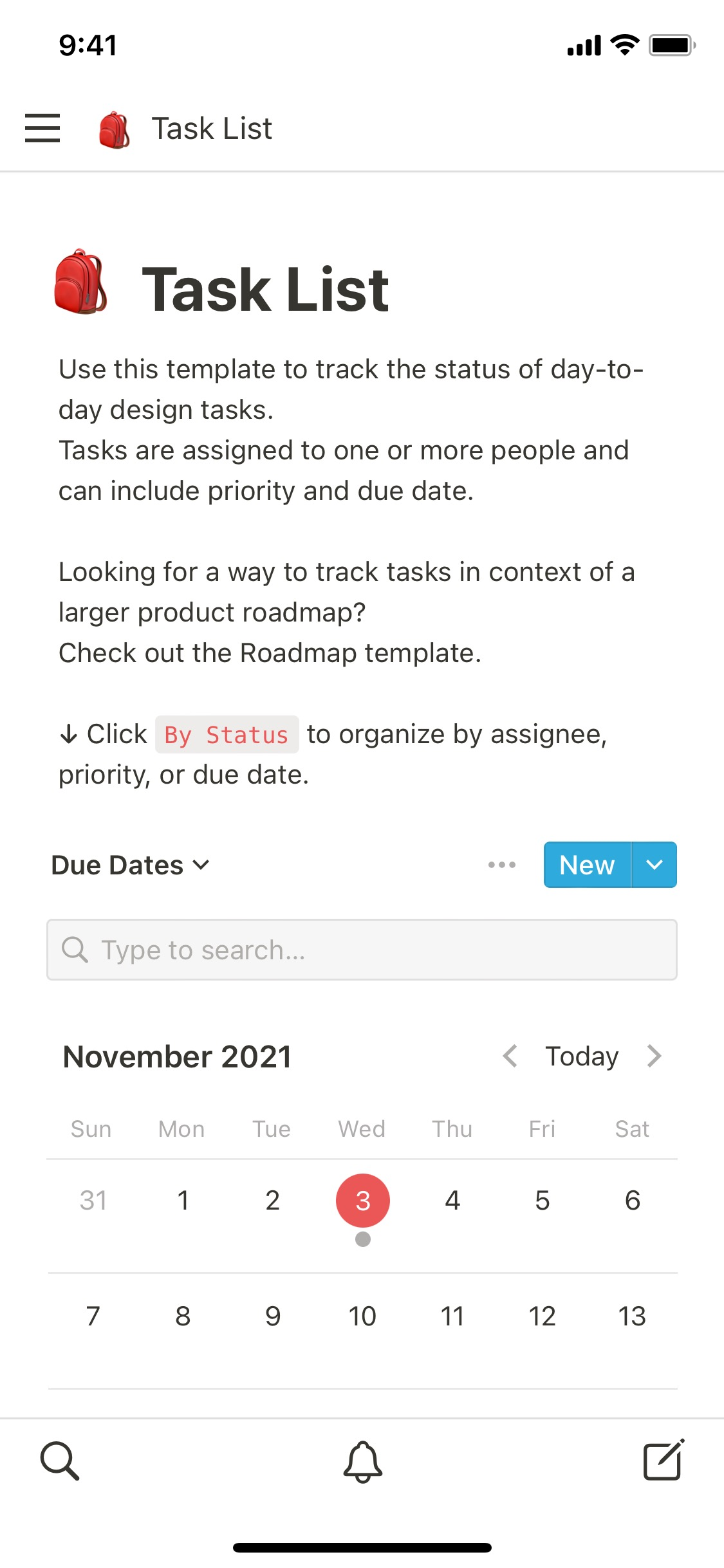The image is a screenshot from a smartphone. The top left corner displays the time, 9:41, while the top right corner shows a fully charged battery icon. Below these indicators, the layout consists of four distinct sections. 

Prominently featured in the upper part is an image of a red backpack, accompanied by the title "Task List." A light gray line separates this area from the main content below. Once again, the red backpack icon and the "Task List" title, now in bold black letters, are presented.

The subsequent text reads: "Use this template to track the status of day-to-day design tasks. Tasks are assigned to one or more people and can include priority and due date. Looking for a way to track tasks in context of a larger project roadmap? Check out the roadmap template." An arrow icon is shown below, prompting users to sort tasks by various criteria: assignee, priority, or due date. The phrase "By status" is highlighted in red text.

Further down, the screenshot features a calendar for November 2021, with Wednesday the 3rd circled in red and a small gray dot beneath the date.

At the bottom of the screen, three icons are displayed: a magnifying glass, a bell, and a thin black line marking the very bottom edge of the page.